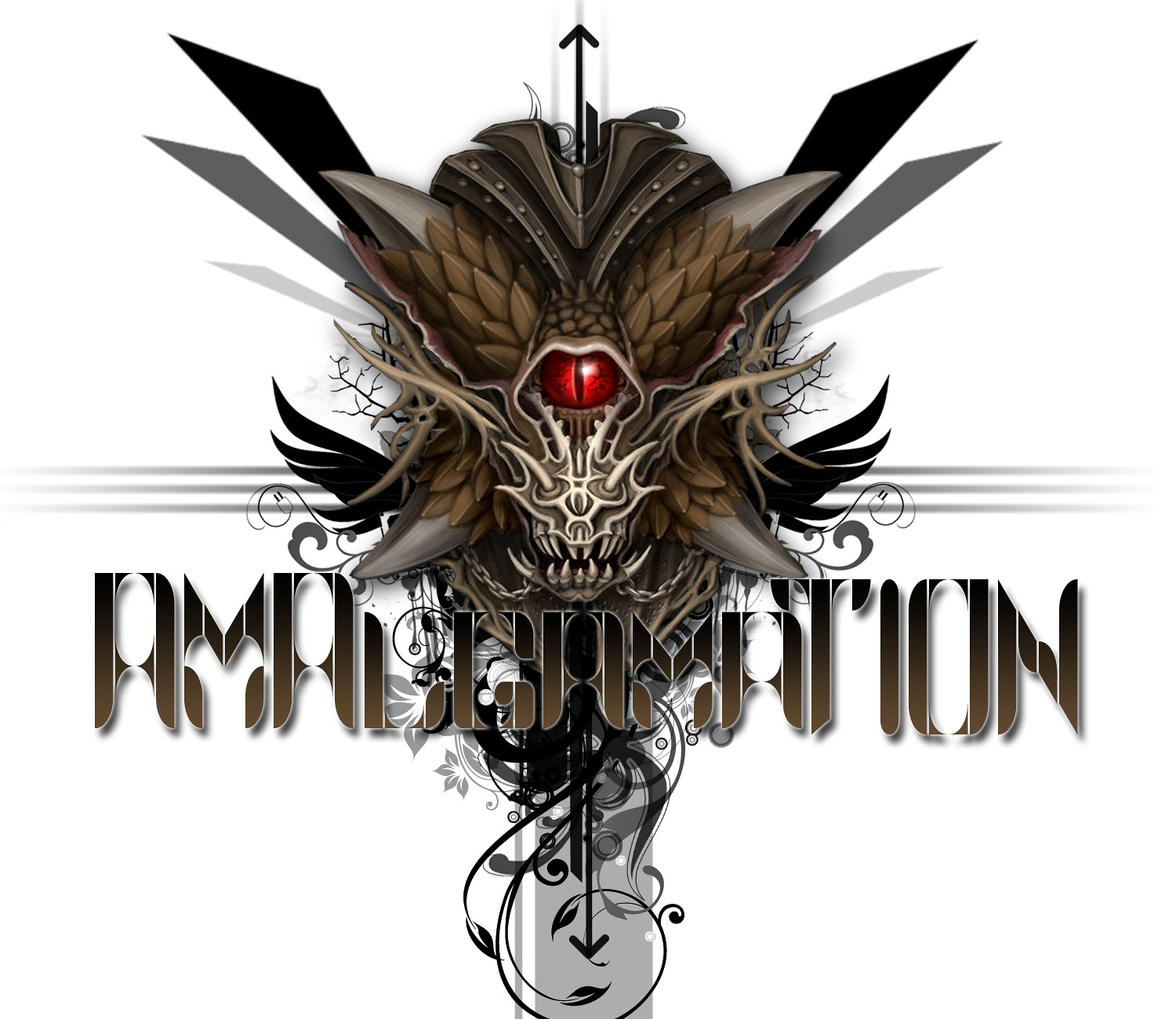The digitally created image, devoid of any border or frame, features a foreboding and intricate creature at its center. This creature has a singular, large red eye reminiscent of a snake’s, positioned above a defined jawline with a partially open mouth filled with jagged teeth. The nose area features sharp, horn-like nostrils. Framing the face are brown, feather-like structures interspersed with black and gray spikes, as well as gray, angled tentacle-like appendages extending from either side of the head. Above the creature’s head, darker brown tentacles emerge. Below the chin, a winding black strand adorned with intricate scrolls and an arrow pointing downward is visible. Across the lower part of the image, difficult-to-read text, possibly spelling "AMALGAMATION," blends into the background due to its broken and similarly colored font. The composition is further accented by faint gray lines extending horizontally and vertically, creating a subtle cross pattern behind the creature.